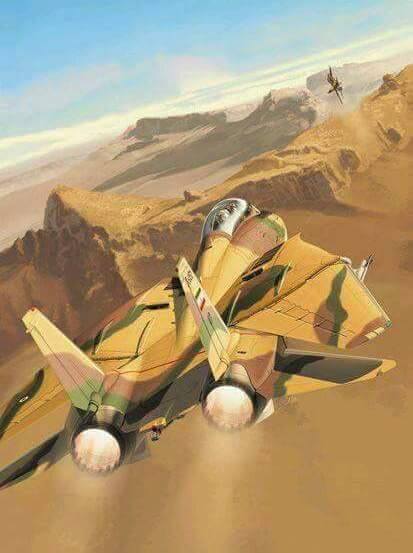The image depicts an animated scene of two camouflage-colored military jets set against a backdrop of dirt hills and mountains with a blue sky partially covered by white clouds. The jet in the foreground, marked by its distinctive double exhausts releasing smoke or steam, indicates rapid movement. The second jet is positioned ahead, appearing to execute a maneuver to its side, suggesting either an attack or training exercise. The aircrafts sport a mix of blue, black, dark brown, and yellowish-brown camouflage, though the cockpit details are indistinct. The animated and somewhat stylized nature of the drawing adds an abstract quality, making it difficult to capture finer details, and there is no name or signature visible in the photo.